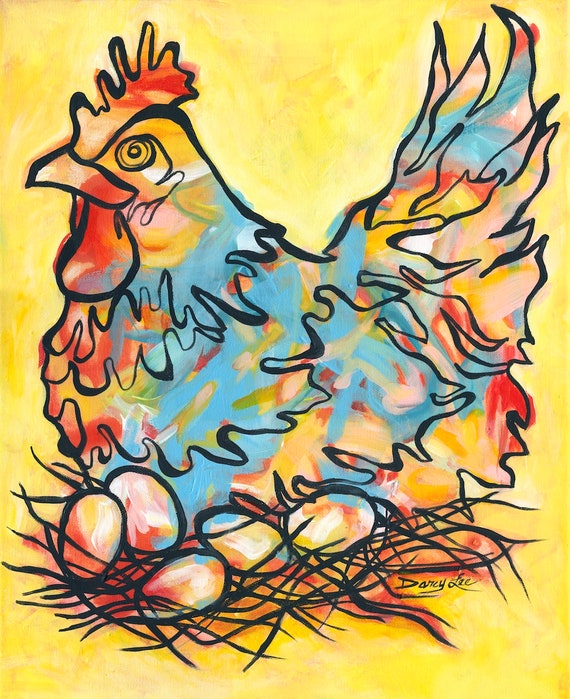This vibrant watercolor painting by Darcy Faye (also referred to as Darcy Lee in some comments) depicts a hen sitting on a nest of five multicolored eggs. The art style is modern and avant-garde, featuring a striking use of colors that blend realism with creativity. The hen is primarily illustrated in shades of blue, accented with touches of yellow, orange, red, and green swirls. The background is a swirling mix of lighter to mid-color yellows with textured details and hints of white and brown. The hen, outlined in black, is positioned in profile facing to the left, with its red comb prominently visible. The nest below the hen comprises black brush strokes, adding a striking contrast to the overall composition. This piece captures the eye with its dynamic colors and whimsical portrayal of a traditional farm scene.